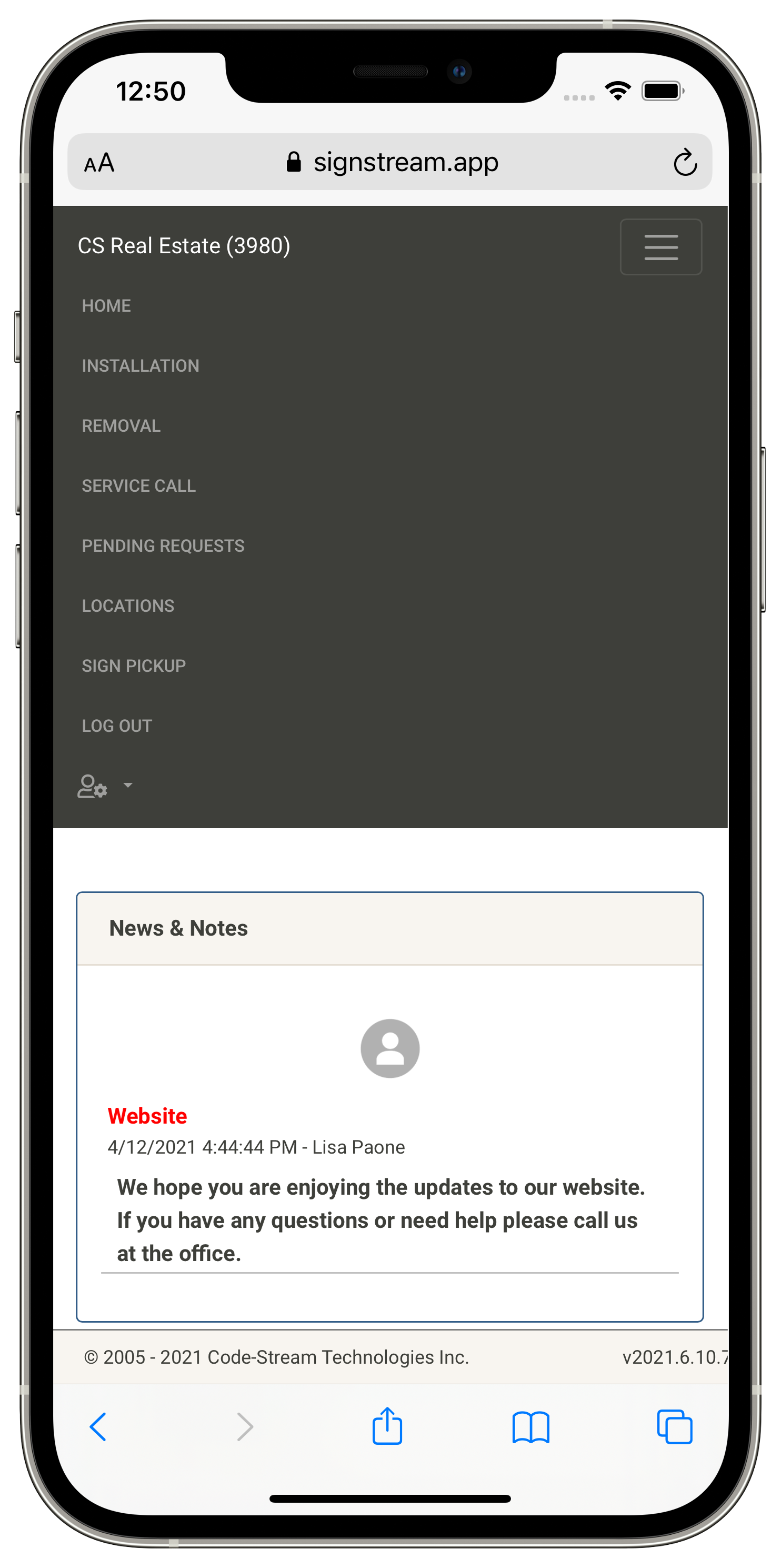A detailed close-up image of a smartphone is displayed, highlighting more than just the screen—it showcases the entire device. In the top-left corner of the phone's screen, the time reads 12:50, though it's unclear whether it's a.m. or p.m. The status indicators show decent internet reception and a full battery. The browser URL at the top indicates a secure site, "stream.app," featuring options to refresh the page and adjust font settings.

Below the browser bar, the main screen displays a black background with "CS Real Estate 3980" in white text. To the right of this text, there is a hamburger menu icon for accessing additional options. Underneath this section, there are several menu items listed in gray text against the black background: "Home," "Installation," "Removal Service," "Call," "Pinning Requests," "Location," "Sign Pickup," and "Logout."

The lower part of the screen transitions to a large white area. Here, a sub-section is visible with the header "News and Notes" featuring a placeholder avatar image with no content inside it. Left-justified in red text, a message reads, "Website April 12th, 2021 at 4:44 p.m." Below this date and time, the message from Lisa states, "We hope you're enjoying the updates to the website. If you have any questions or need help, please call us at the office," indicating a proactive customer satisfaction check.